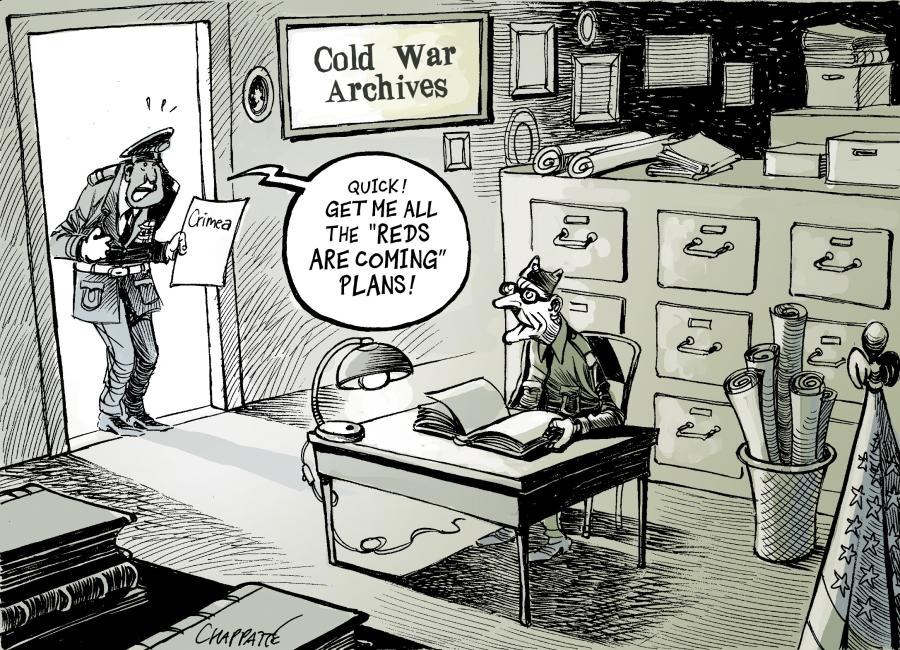In this black and white or sepia-toned political cartoon, the setting is a military office, highlighted by a sign on the wall that reads "Cold War Archives." An elderly man with black glasses, who appears slightly sleepy, is seated at a metal desk. He's dressed in a Vietnam War-style uniform and has an open book illuminated by a lit desk lamp. Beside him is a large filing cabinet with nine visible drawers and several scattered papers. In the bottom right corner, part of an American flag can be seen.

Bursting through an open door to the left, a desperate-looking officer in a formal military uniform, complete with a hat, urgently holds out a white piece of paper labeled "Crimea." With a frantic expression and an open mouth, he exclaims, "Quick, get me all the 'Reds are coming' plans!" as he looks directly at the seated man. The wall near the door also features a poster labeled "Cold War Archives," reinforcing the historical context of the scene.